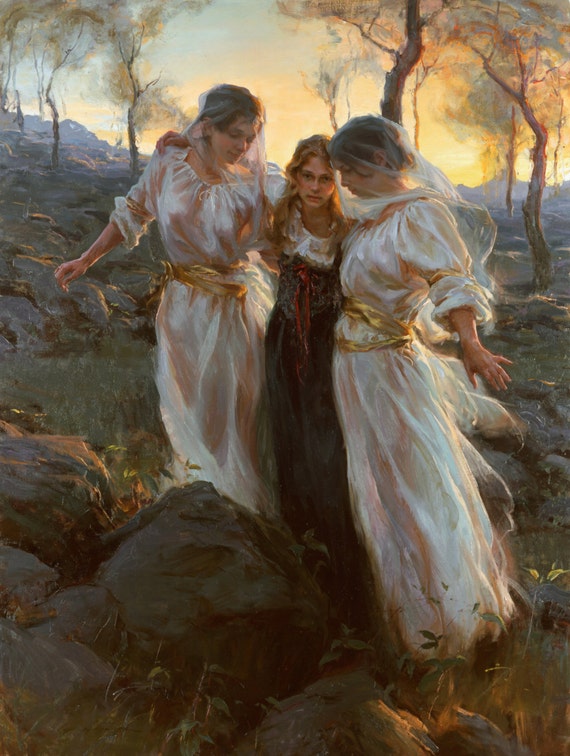This painting, possibly a computer-generated image, showcases a detailed scene with three female figures in a mystical forest setting under a cloudy sky. Two women, dressed in long, flowing white gowns with golden sashes around their waists, necklines, and upper arms, stand on either side of a younger girl. The women have short, dark hair adorned with clips, visible beneath semi-transparent white veils. Their arms are gently extended, as if gliding or offering support to the girl in the middle. The younger girl appears lost and confused, wearing a black dress with a red bow and a layered white top. Her light brown hair cascades around her shoulders. The scene includes whimsical elements, with lush plants growing on rocks to the left and a smattering of trees in the background, along with tall grass and more stones, adding to the ethereal atmosphere. The two women in white, possibly representing guardian angels, seem to be guiding or comforting the girl in this serene yet enigmatic woodland.